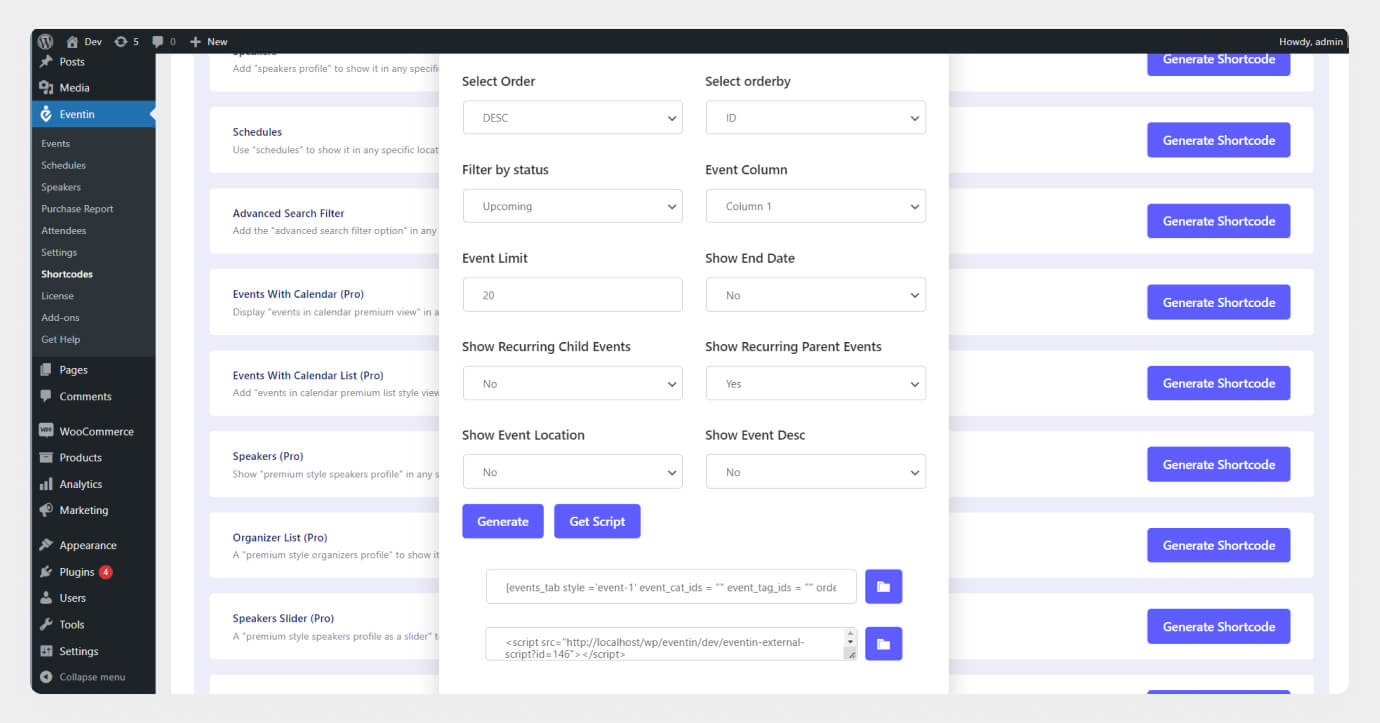The screenshot, displayed in landscape mode, appears to be taken from a laptop showing a webpage, surrounded by a light gray border. The primary focus of the image is the website interface.

At the very top of the page, a black stripe stretches from the upper left-hand corner to the upper right-hand corner. On the left side of this stripe, there is a circular "W" logo, presumably representing WordPress, followed by the text "DEV" and a number "5". Additionally, there is a plus sign for adding new content. The upper right-hand corner features the greeting "Howdy Admin".

The webpage is divided into multiple columns, with the leftmost column featuring a black background. This column lists various sections, including:
- Posts
- Media
- Event In
- Events
- Schedules
- Speakers
- Purchase Report
- Attendees
- Settings
- Shortcodes
- License
- Add-on
- Get Help

Beneath this list, an even darker section includes:
- Pages
- Comments
- Woo (Commerce)
- Products
- Analytics
- Marketing
- Appearance
- Plugins (with a notification badge indicating "4")
- Users
- Tools
- Settings
- Collapse Menu

Notably, the "Event In" section is highlighted in blue, indicating it is currently selected, which explains the pop-up menu visible on the screen. This pop-up menu has a white background and functions as a form with several options:
- Select Order
- Select Order By
- Filter By Status
- Event Column
- Event Limit
- Show End Date
- Show Recurring Child Events
- Show Recurring Parent Events
- Show Event Location
- Show Event Desk

There are two buttons labeled "Generate" and "Get Script", followed by a series of scripts that can be copied. Behind this pop-up form, numerous rows are visible, each featuring purple "Generate Shortcode" buttons on the right side.